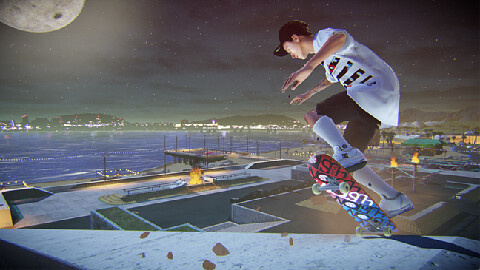A dynamic screenshot from a skateboarding video game depicts an athlete mid-action at a sprawling skatepark. The skateboarder, clad in a black hat, white t-shirt, black shorts, long white socks, and white shoes, has just ascended a towering ramp on the right side of the scene. Balanced at the ramp's peak, with the skateboard angled upwards, the skater appears poised to execute a flip maneuver and descend back down. The setting occurs at nighttime, with a captivating view of the ocean on the left and the distant city lights illuminating the horizon. The scene is further enriched by a prominent full moon positioned in the upper left-hand corner of the sky.